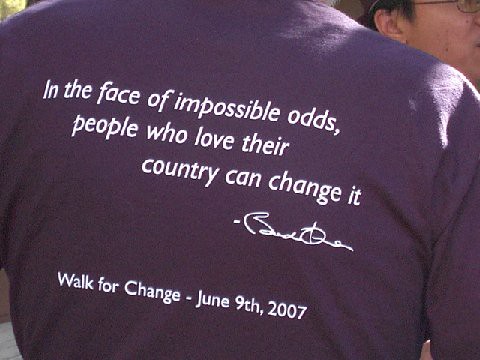The image captures the back of a purple t-shirt, prominently displaying a white print with the quote: "In the face of impossible odds, people who love their country can change it." Below the quote is a signature, indicated to be Barack Obama's, and further down, the text reads: "Walk for Change, June 9th, 2007." The t-shirt takes up most of the frame, but on the right side of the image, part of a person's face with dark hair and black-framed glasses is visible. This half-face suggests the presence of others, likely at an event supporting a cause indicated by the "Walk for Change." Light is shining on the right shoulder of the person wearing the t-shirt, highlighting the details of the shirt’s message.